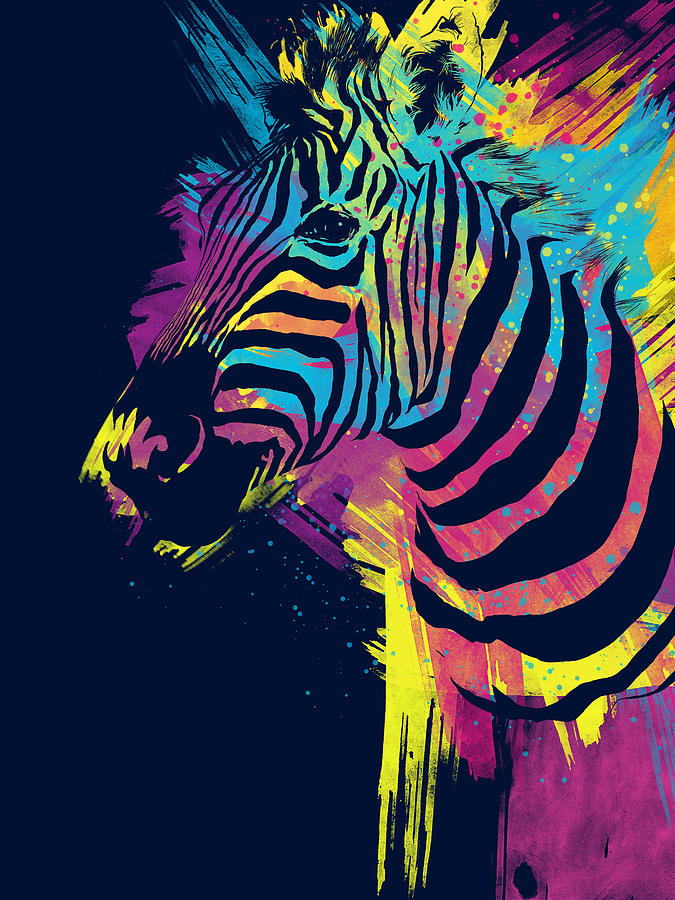The image is an abstract digital illustration of a zebra's head and neck, against a dark blue or black background. The zebra is depicted with its face turned slightly to the left. What makes this zebra unique is the vibrant and chaotic mix of colors where one would normally expect white. The zebra's face features black stripes with patches of vivid purple, blue, and yellow. Its nose is a striking bright purple, while the upper part of its head is painted in bright blue, and there are patches of yellow randomly placed around the face. The neck area primarily displays a bright pink with blue dots, along with yellow areas seemingly dripping off. Only one eye, fur, and a single pointed ear are visible, with the rest of the zebra’s body not depicted. The overall impression is as if the artist threw various bright colors onto a canvas, outlined the black stripes of the zebra, and left the colors to form a seemingly disordered, yet artful, composition.